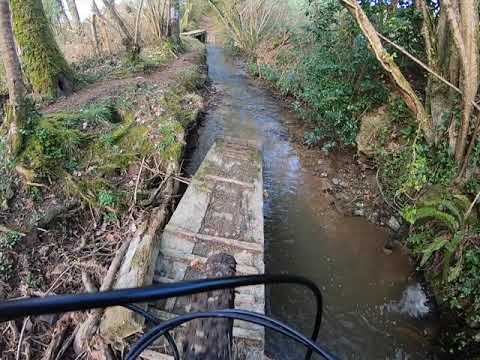The image showcases a square photograph of a narrow, brown stream cutting through a dense wooded area. The stream is flanked by earthy mounds and patches of greenery, including grass, shrubs, and moss-covered tree trunks. In the foreground, a weathered, brown wooden railing, likely a part of a staircase, extends from the lower left heading across and downward to the center. Adjacent to the railing, towards the bottom left, lie some twigs and possibly a bicycle wheel entangled with black brake cables. The water flows gently through the scene, characterized by its opaque brown and grayish hues. Above the stream, thin tree branches weave intricately, with the thickest branch in the upper left corner adorned with bright green moss. The upper right corner reveals a small, bright patch of sky, denoting daylight. A rugged, mossy wooden platform appears as though it is lowering into the creek. The entire area, bathed in natural light, evokes a serene yet somewhat untamed woodland atmosphere.